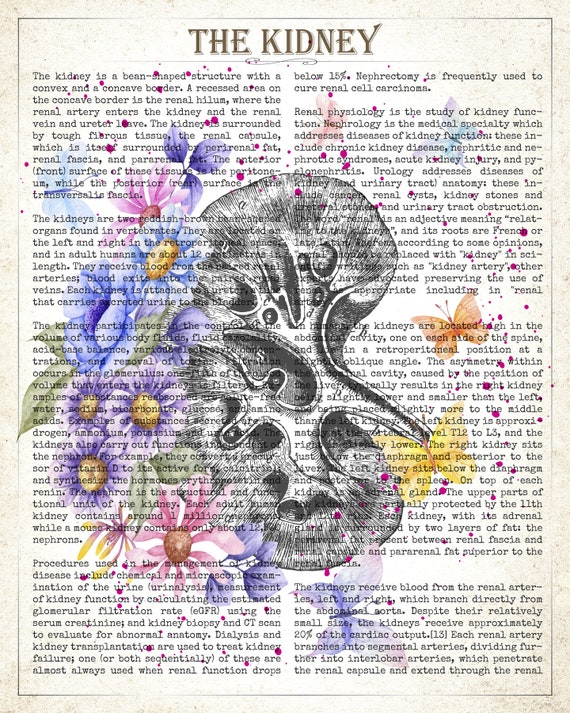This image features a page from a book with a creamy white background and a thin black border. At the top, in large, capitalized black letters, is the title "THE KIDNEY." The page is filled with text describing what the kidney is and its functions. Superimposed on this text are colorful, detailed drawings, including leaves and various flowers—pink, blue with yellow centers, and multiple purple flowers with golden centers. Green leaves are also scattered throughout the page. Additionally, there are butterflies: a larger yellow one, an orange one, and a translucent butterfly with blue and pink hues. A black and white drawing, seemingly a cross-section of a kidney, is also present among the illustrations. The artistic elements make it difficult to read the text fully, giving the impression that someone transformed a page from a book into an intricate piece of mixed-media art.